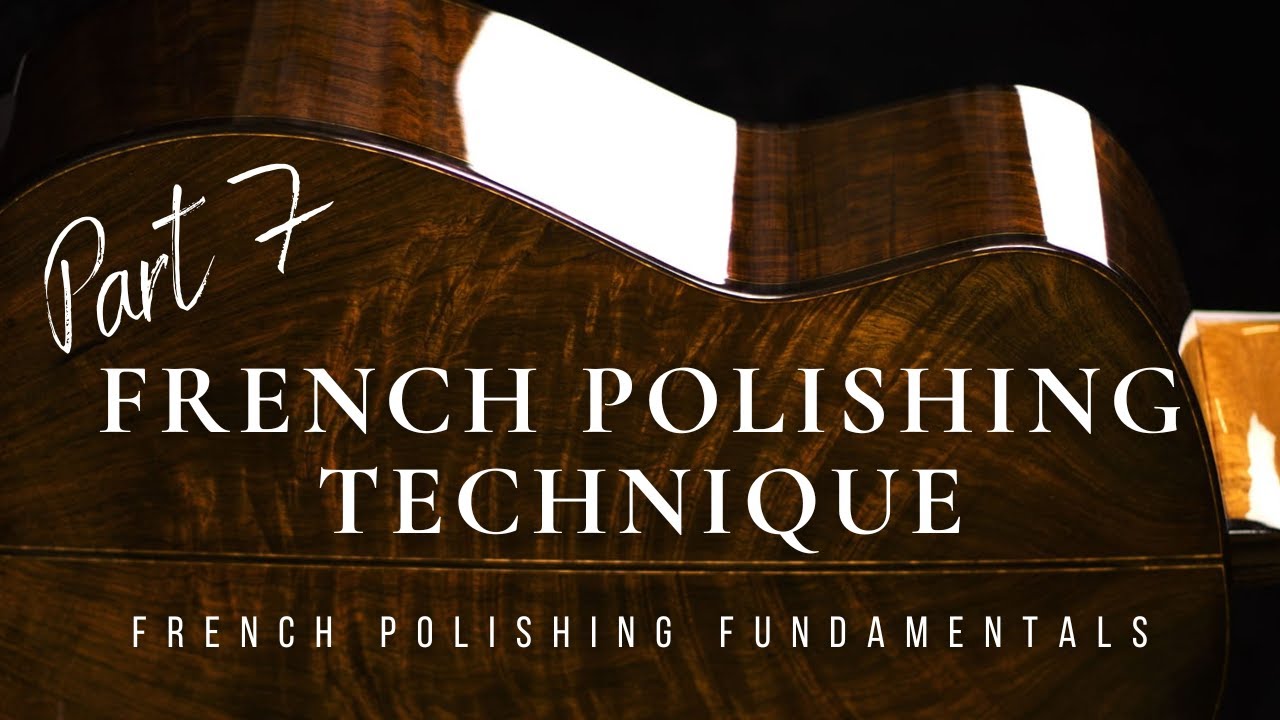This image, part of a web series, is titled "Part 7: French Polishing Technique" with a subtitle "French Polishing Fundamentals." It prominently features the back of a cello with a lustrous vinyl finish on the wooden surface. The cello, angled slightly, allows a partial view of its shiny side, which reflects the light source emanating from the right side of the image. The neck of the cello extends gracefully to the right. Set against a stark black background, the white lettering of the title and subtitles stands out clearly on the left side of the image. The light from the right highlights the elegant contours and polished surface of the instrument, emphasizing the craftsmanship of the French polishing technique.